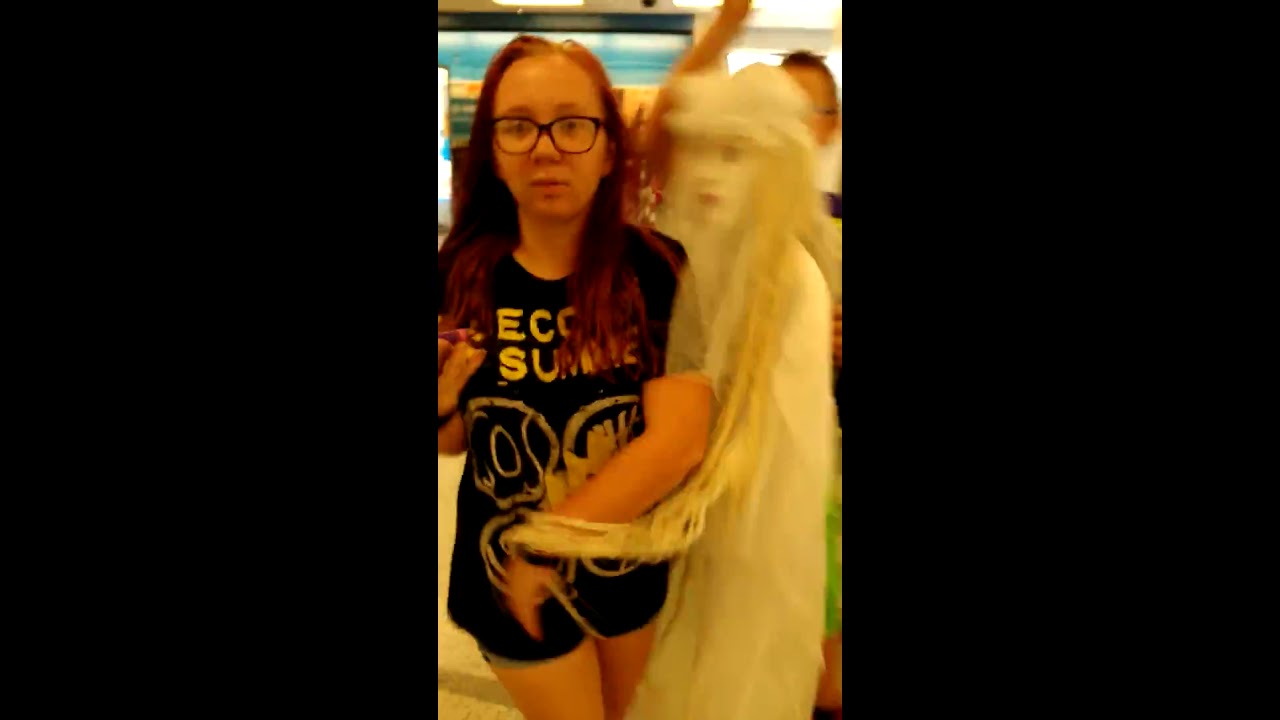In the center third of the image, a young, light-skinned female with long reddish-brown hair and black-rimmed eyeglasses is looking towards the camera. She has a distinct oval face with a large forehead and is dressed in a black T-shirt with white text that seems to spell out "summer," possibly including "ECC" and the number "86." She is also wearing blue jean shorts. Beside her, to her right, stands a ghost-like mannequin with pale white skin, long white hair, and a white bonnet, adorned in a long white gown. The mannequin appears to be interacting with the girl, as its arm is wrapped around her left wrist. The background features a man with his hand raised up. The left and right thirds of the image are bordered with very thick black frames embellished with metallic sparkles, which contrast starkly with the clear central portion of the photograph.